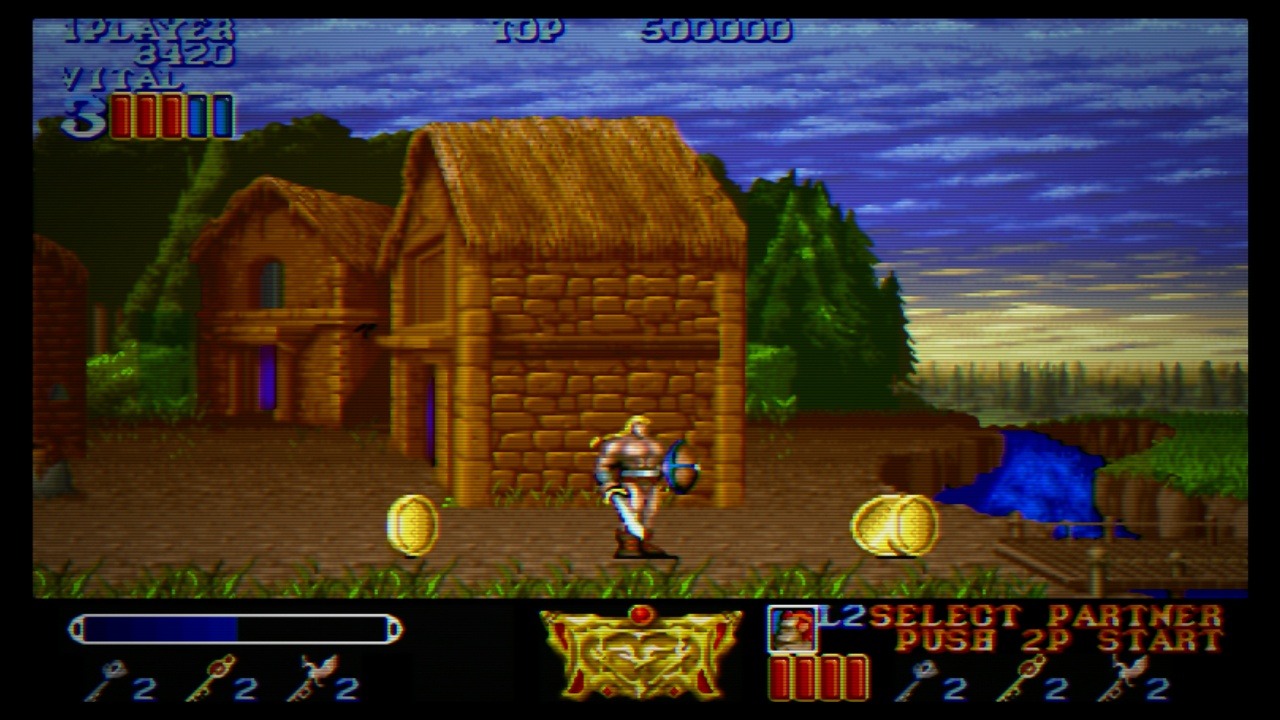This screenshot from a retro 90s-era video game, potentially resembling SNES graphics, prominently features a detailed interface and vibrant scene. At the top left, game stats display "One Player" and a score of 3,420. Below this, "Vital 3" is visible alongside a meter with three red rectangles and two blue rectangles. The bottom section showcases tool icons and alerts reading "Select Partner" and "Push 2P Start."

The central figure in the image is a white-skinned man clad in only a brown loincloth, brown boots, and a metal sword in his right hand. His left arm wields a wooden shield with blue stripes. He has long blonde hair, and stands amidst large golden coins scattered on the ground. 

The background sets a rustic scene with stone houses featuring straw roofs, a flowing river, and dense trees. Additionally, a brown bridge arches over the river at the bottom right, while the sky overhead is a vibrant blue with scattered white clouds.